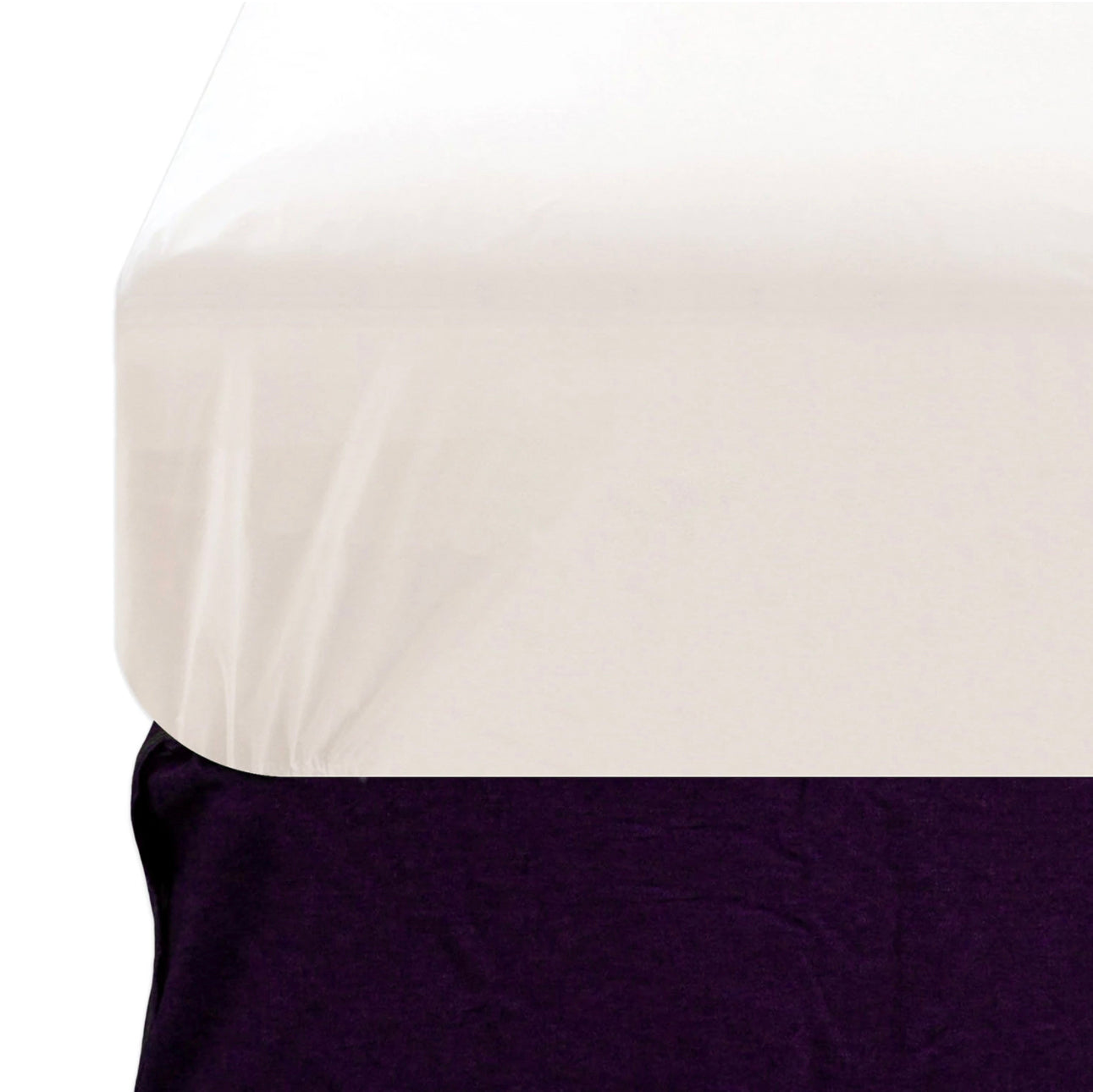The photograph showcases a detailed close-up of a bed, focusing on the corner where a white fitted sheet is snugly secured over a mattress. The mattress, which appears to have a slight sheen, suggesting it might be made of a satin-like material, rests atop a base that is black in color. The image, taken at an angle, illustrates the distinct cuboid shapes of both the mattress and the base, with the mattress exhibiting rounded corners for added detail. Shadows and highlights on the sheet and base suggest depth but add no additional colors, maintaining a monochromatic theme of black and white throughout the composition. The simplicity and detail of the shot, likely intended for a product listing on a retail site, emphasize the secure fit of the sheet on the bed's corner, possibly to market the quality and fit of the sheet set.